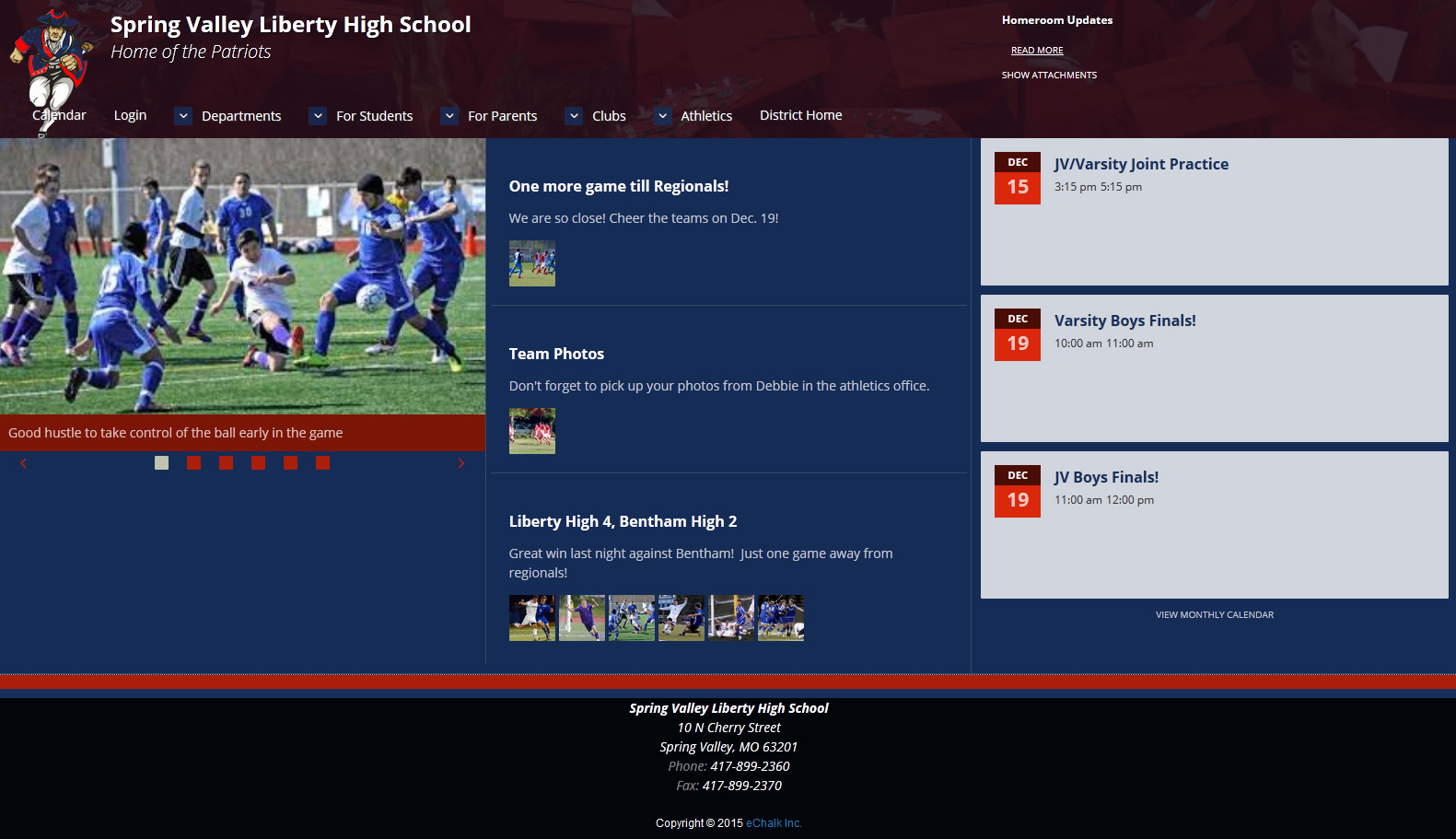This website screenshot features a clean, black background that frames the content at both the top and bottom. On the top left, there's an eye-catching cartoon mascot dressed in historical attire reminiscent of the 1700s, symbolizing the school's rich heritage. Next to the mascot, the header prominently reads "Spring Valley Liberty High School" in white, capitalizing the first letter of each word. Beneath this title, the tagline "Home of the Patriots" proudly sits.

The navigation bar provides a variety of options: Calendar, Login, Departments, For Students, For Parents, Clubs, Athletics, District, and Home. On the opposite side, the menu includes quick links such as Homeroom Updates, Read More, and Chats Run.

Further down, a standout blue section features an action-packed image of athletes on a soccer field. Below the image, a vibrant red banner headlines "Good Hustle: Tips and Tricks to Take Control of the Ball Early in the Game." Adjacent to this is an announcement about an upcoming game: "One more game until regionals - Team Photos: Liberty High 4, Bentham High 2."

The bottom section is organized with individual images and key event dates:

- December 15: JV & Varsity Joint Practice
- December 19: Varsity Boys Finals
- December 19: JV Boys Finals

Specific times for these events are also provided, ensuring that visitors have all the pertinent details at their fingertips.